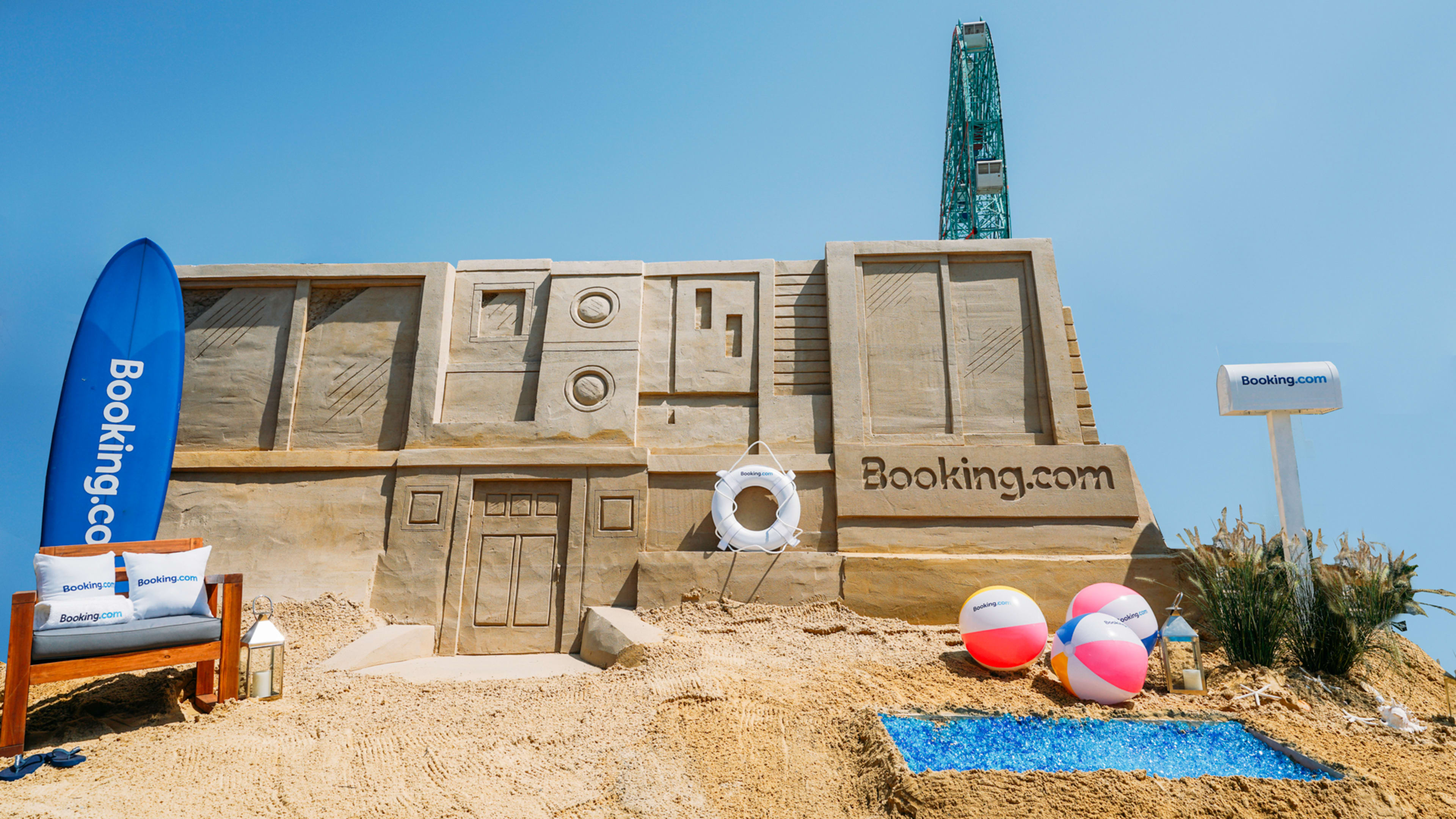The image is a promotional setup for Booking.com, featuring a sandcastle-like house adorned with various beach-themed details. Centered prominently is a white life preserver. To the bottom left, three beach balls in shades of pink and white lie near a small blue sand-filled hole resembling a pool. On the right side, there is a white mailbox with "Booking.com" written on it, positioned above a tiny shrub. Adjacent to the house is a blue surfboard, and an orange chair with white pillows also bearing the Booking.com logo. Rising at the top right of the sandcastle is a Ferris wheel structure. The background is a clear, blue sky, suggesting a sunny beach day. The entire tableau combines elements of a modern building with playful, beach-related accessories, all rendered in soft hues of tan, white, pink, yellow, blue, green, and light brown, encapsulating a whimsical yet promotional scene for Booking.com.